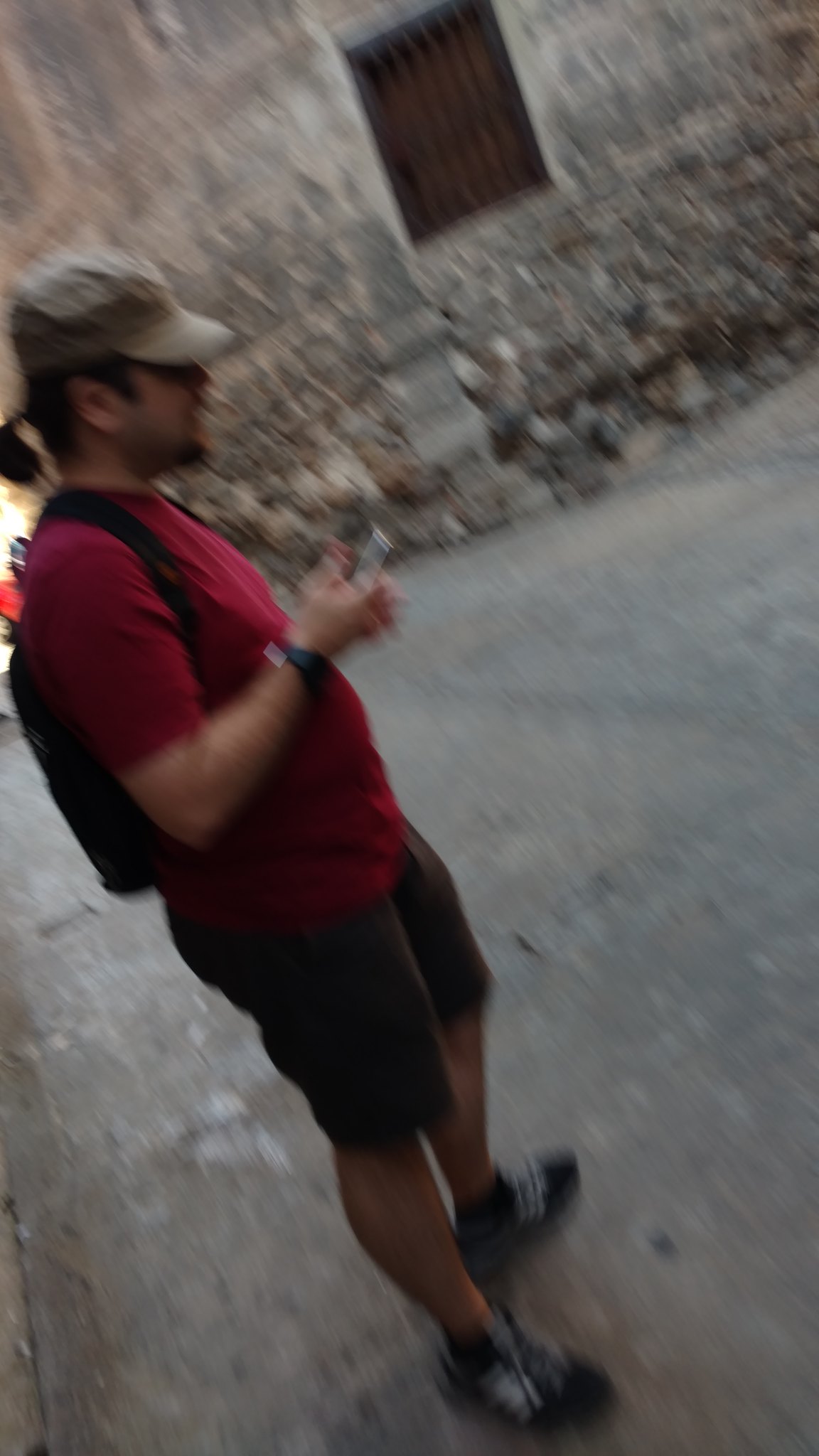In this daytime photograph, although extremely blurry and low resolution, the scene is discernible. A young man stands diagonally on a concrete path or road, his feet pointing towards the lower right corner of the image and his head towards the upper left. Captured from a side view, he is dressed in dark shorts, a vibrant red t-shirt, and a khaki baseball cap that reveals a dark-haired ponytail at the back. The man has a beard and mustache, and wears glasses. On his wrist is a black watch, and he holds what appears to be a cell phone in his hand. His footwear consists of tennis shoes. 

Behind him looms an old stone building with a patchwork of multi-shaped stones, suggesting it may be ancient ruins, potentially dating back hundreds or even thousands of years. The stone structure varies in color from gray to cream and light camel, adding to its historic aura. The bottom of the building appears crumbled, contributing further to its aged and worn appearance. An open window punctuates the weathered wall, adding a focal point to the background.